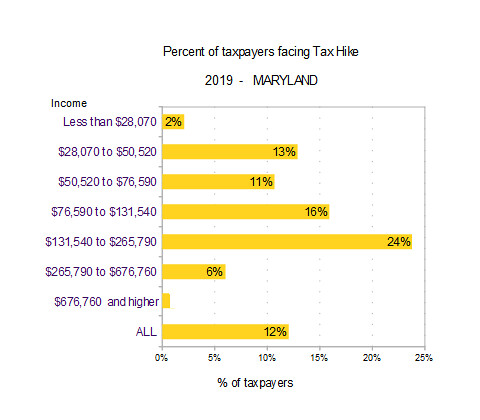The image is a yellow-bar chart titled "Percent of Taxpayers Facing Tax Hike 2019 - Maryland," centrally positioned, likely from a news website. The vertical y-axis represents different income brackets, starting from the top at "less than $28,070" and segmented as follows: "$28,070 to $50,520," "$50,520 to $76,590," "$76,590 to $131,540," "$131,540 to $265,790," "$265,790 to $676,760," and "676,760 and higher." The final category simply labeled "all." The horizontal x-axis shows the percentage of taxpayers, marked in 5% increments from 0% to 25%. The chart's bars display the following percentages for each income bracket from top to bottom: 2%, 13%, 11%, 4%, 16%, 5%, 24%, 6%, with the penultimate bar being quite low at approximately 1%, and the final "all" bar indicating 12%. The image features a clean, simple color scheme of white, black, and yellow.